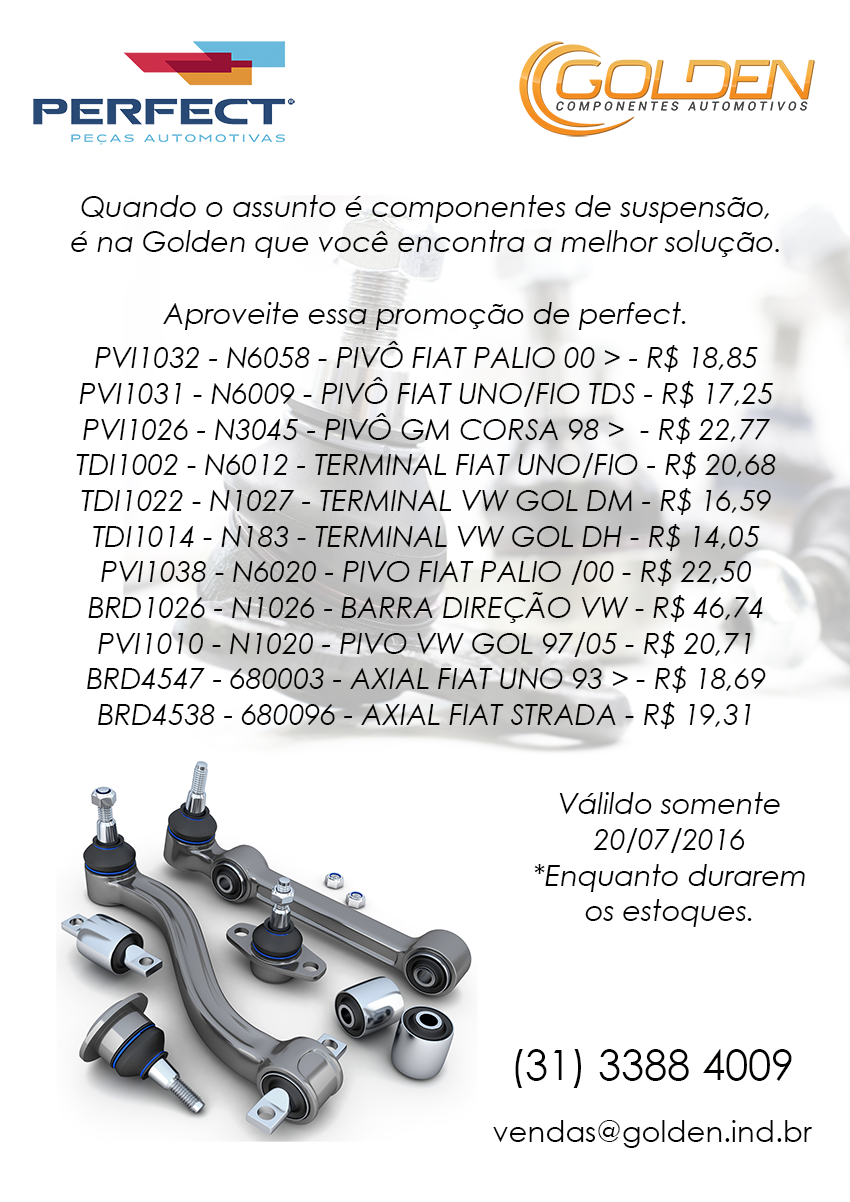This is a vertically aligned rectangular promotional flyer primarily in Portuguese, featuring a price chart for various automotive or machining parts. The top left corner displays the logo "Perfect Pecas Automotivas" in dark blue and light blue font, with a design of staggered rectangles in blue, red, and orange above it. The top right corner features another logo with "Golden" in gold letters and "Componentes Automotivos" in black beneath it. 

The flyer has a white background with a light gray section in the middle, overlaid with black text describing the products. It includes a centered promotional message stating, "Quando o assunto é componentes de suspensão, é na Golden que você encontra a melhor solução. Aproveite esta promoção da Perfect." Below this, there are approximately ten lines listing various parts with their descriptions and prices.

In the bottom left corner, the flyer depicts several screws and machine parts, including levers and switches, with additional accessories scattered around. The bottom right corner contains a phone number, "3133884009," and an email address, "vendasatgolden.ind.br," indicating the flyer is for a Brazilian market.